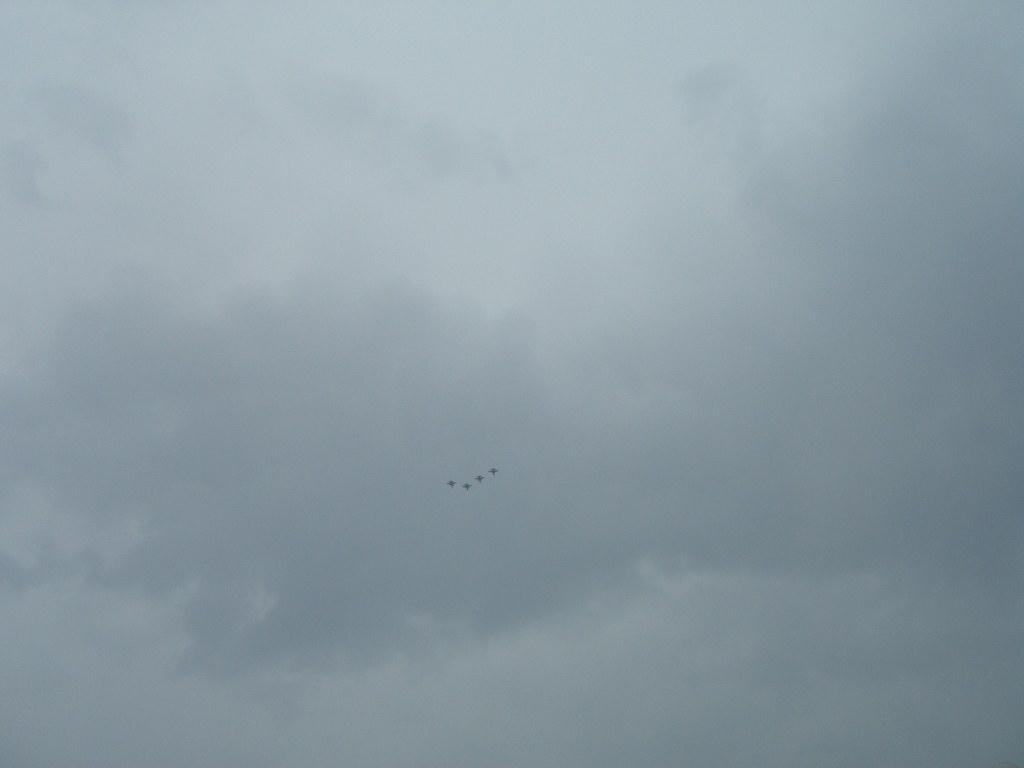This photo captures a dramatic, overcast sky with varying shades of gray clouds that dominate the scene. Sunlight attempts to pierce through, but is mostly muted and filtered by the dense cloud cover. Positioned midway through the image and slightly to the left are four dark objects, tightly aligned side by side. They are distant and ambiguous — seemingly small plus signs against the vast cloud backdrop — making them resemble either birds or airplanes in formation. Their coordination is reminiscent of the Blue Angels' military acrobatics, flying in a V-shaped pattern. The absence of other reference points in this monochromatic gray expanse leaves their true nature and direction uncertain, adding to the intriguing and somewhat mysterious atmosphere of the photograph.